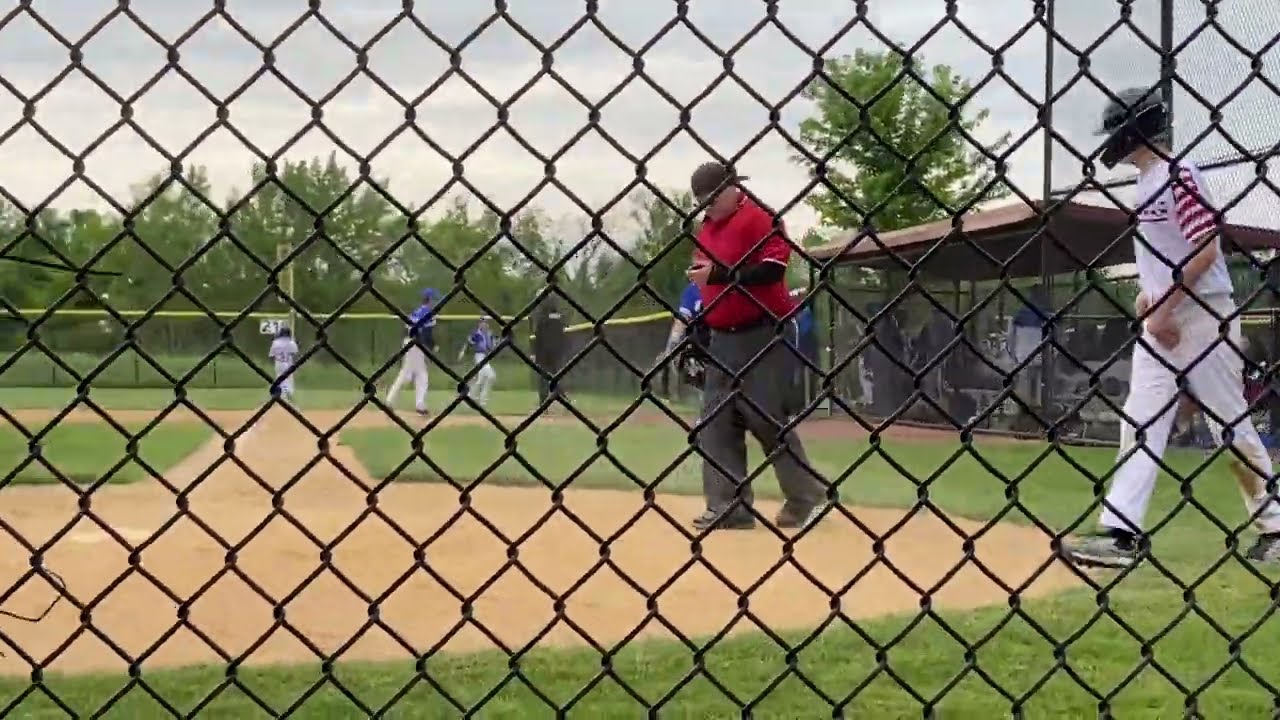This daytime color photograph, taken from behind a black chain-link fence in landscape orientation, captures a detailed scene of a baseball field. The perspective suggests the photographer is either sitting or crouching, as the chain-link fence dominates the foreground and the players appear taller.

On the right-hand side, a player dressed in a white jersey with red and blue horizontal stripes on the sleeves, white pants, and a black helmet is walking leftward across the grass. Parallel to him, on the dirt portion of the field, an umpire wearing a red shirt, long-sleeved black undershirt, dark pants, and a backwards black cap, is engrossed in his cell phone as he walks.

In the background to the right, a partially visible dugout pit is present, with players donning blue jerseys walking towards it. The scene is under a notably gray sky, adding to the realism and representational style of the photograph. Trees encircle the field's backdrop, emphasizing the outdoor setting.